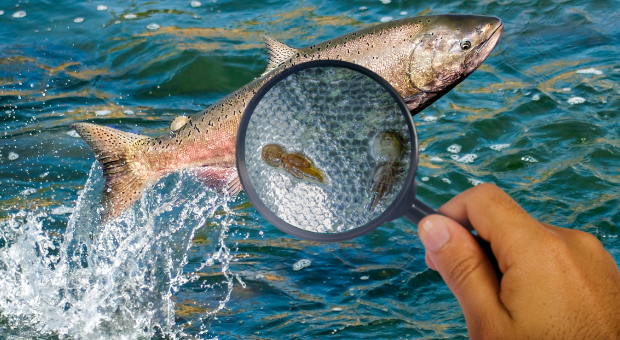In this highly detailed, color photograph, a fish with bronze, beige, and pink tones, measured around 12 inches, is captured in mid-leap from a dynamic, dark blue ocean with white splashes accentuating its jump. The fish, positioned diagonally with its mouth closed and eyes open, displays silvery metallic scales, a small dorsal fin, and a speckled silver and black tail. Overlaid on this scene, a tan-skinned human hand protrudes from the bottom right corner, holding a dark gray magnifying glass. Within the magnifying glass's circular frame, a close-up reveals detailed fish scales with tiny marine creatures attached. However, the image within the magnifying glass and the hand itself are incongruous with the main photograph, likely photoshopped due to mismatched angles and differing color tones. The overall composition artfully attempts to illustrate a microscopic view of the fish's scales but is visually disjointed, highlighting the human intervention in the scene.